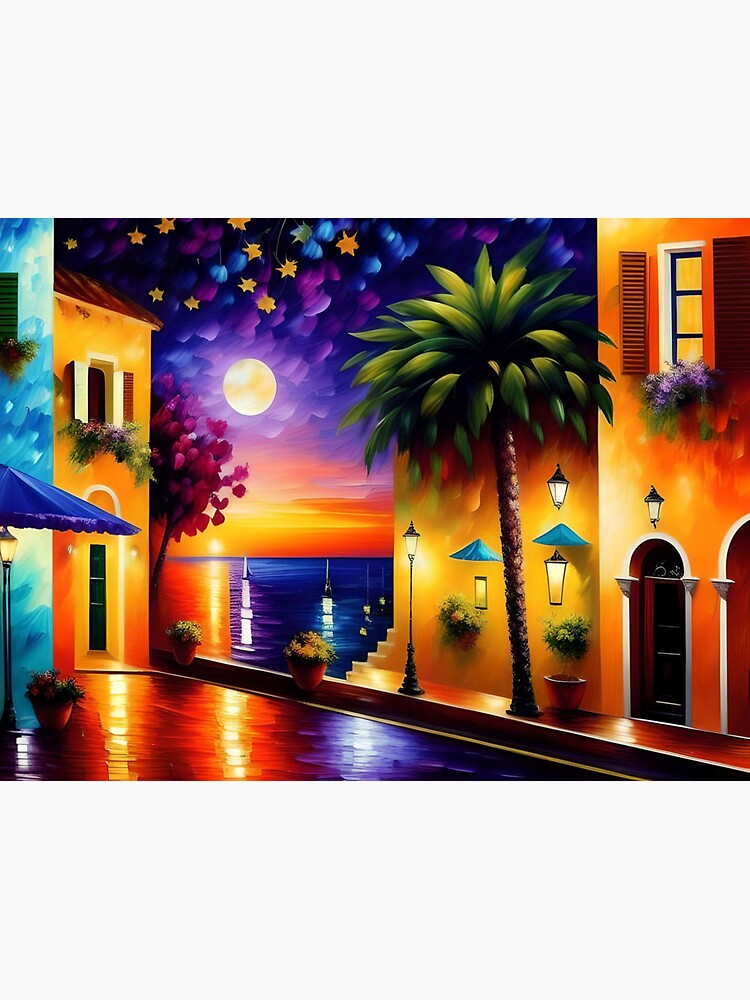The painting is a vibrant and colorful depiction of a Mediterranean or Caribbean-style street at sunset. The scene features a mix of two-story stucco buildings painted in shades of orange, blue, and yellow, adorned with arched doorways and brown wooden windows thrown open. The upper stories are decorated with window boxes brimming with greenery. A large palm tree stands prominently on the right sidewalk, alongside pots of green plants, while a red tree is situated near the left-side building that extends over the water.

Overhead, the sky transitions from deep blues and purples at the top to warm oranges and yellows near the horizon, dotted with golden and blue stars. The full moon is visible above a body of water that reflects its glow, along with the colors of the setting sun. Lanterns with glass panels cast a warm illumination on the cobblestone street below, which also reflects the ambient light. In the distance, a couple of sailboats float on the water, adding to the tranquil, deserted ambiance of this tropically infused Art Deco scene.